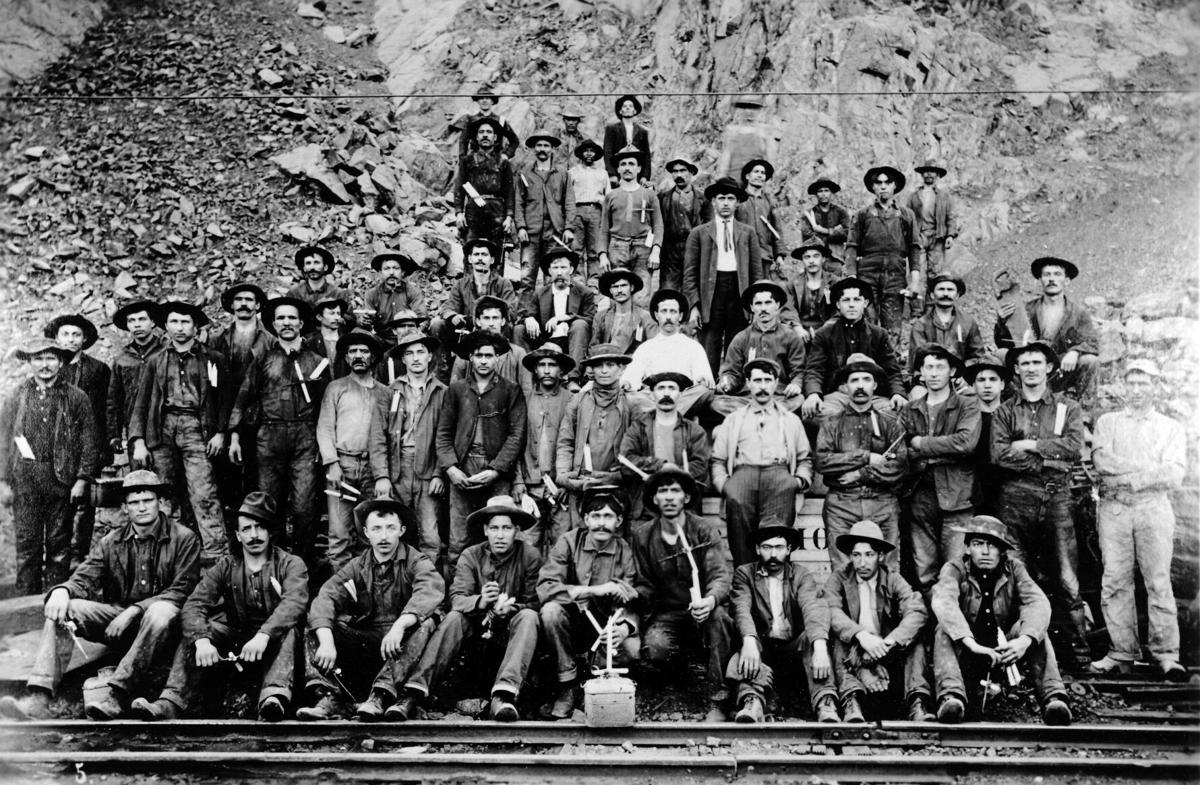This is a rectangular black and white photograph depicting a large group of railroad workers, likely from the mid-19th century in the United States. The workers are predominantly Caucasian men, and they are arranged in several rows on a hillside covered in rocks and rubble, indicative of a recent landslide or excavation. The bottom of the photograph features railroad tracks running horizontally across the image. The men, all wearing hats with brims and dressed in long sleeve shirts and pants, are positioned with the front row sitting down, their feet resting on the tracks. Behind them, additional rows of men are staggered up the rocky incline, making the groups further back appear smaller as they ascend. Some workers are equipped with tools such as saws, while a few in the group are notably wearing jackets and ties. The background of the image showcases a rugged, blasted mountain, adding context to the industrial and manual labor setting captured in the photograph.